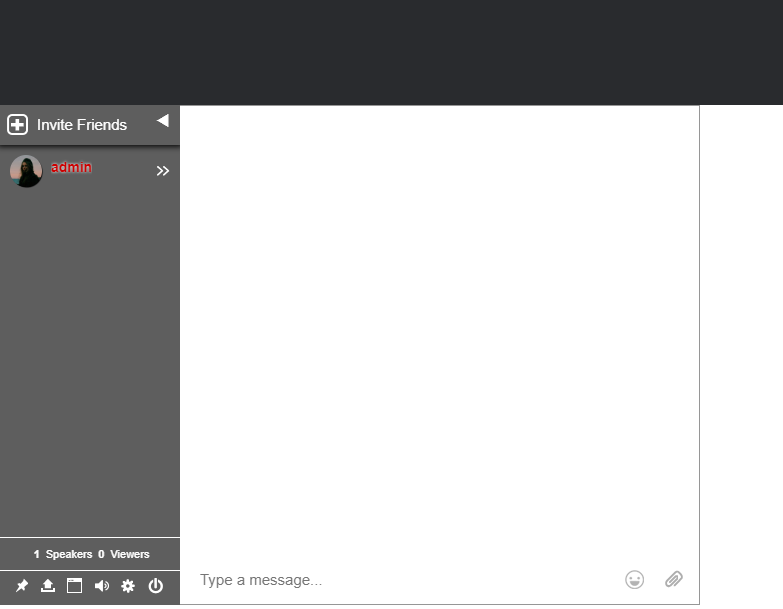Caption: 

A cropped screenshot of a collaboration app interface is displayed. The top part of the interface is dominated by a large, empty black banner. Below this, on the left side, there is a dark gray vertical panel. At the top of this panel, a white plus sign is visible, with the text "Invite friends" centered to the right of it. Adjacent to this text, there is a left-pointing triangle indicating a dropdown menu. 

Further down the panel, a circular profile picture is located on the left, next to the text "admin" written in lowercase red letters. To the right of this, two right-pointing arrows suggest another selection or navigation tool.

At the bottom of the vertical panel, there is text indicating "1 speakers, 0 viewers." Following this, icons for various functionalities are lined up: a pin icon, a send icon, a maximize tab icon, a sound icon, a settings icon, and a power icon.

On the right side of the screenshot, the majority of the page is occupied by a large text box, presumably for main content or chat. At the bottom of this text box, there is a message input field labeled "Type a message." To the right of this input field, there are two small icons: a smiley face for emojis and a paperclip for attachments.